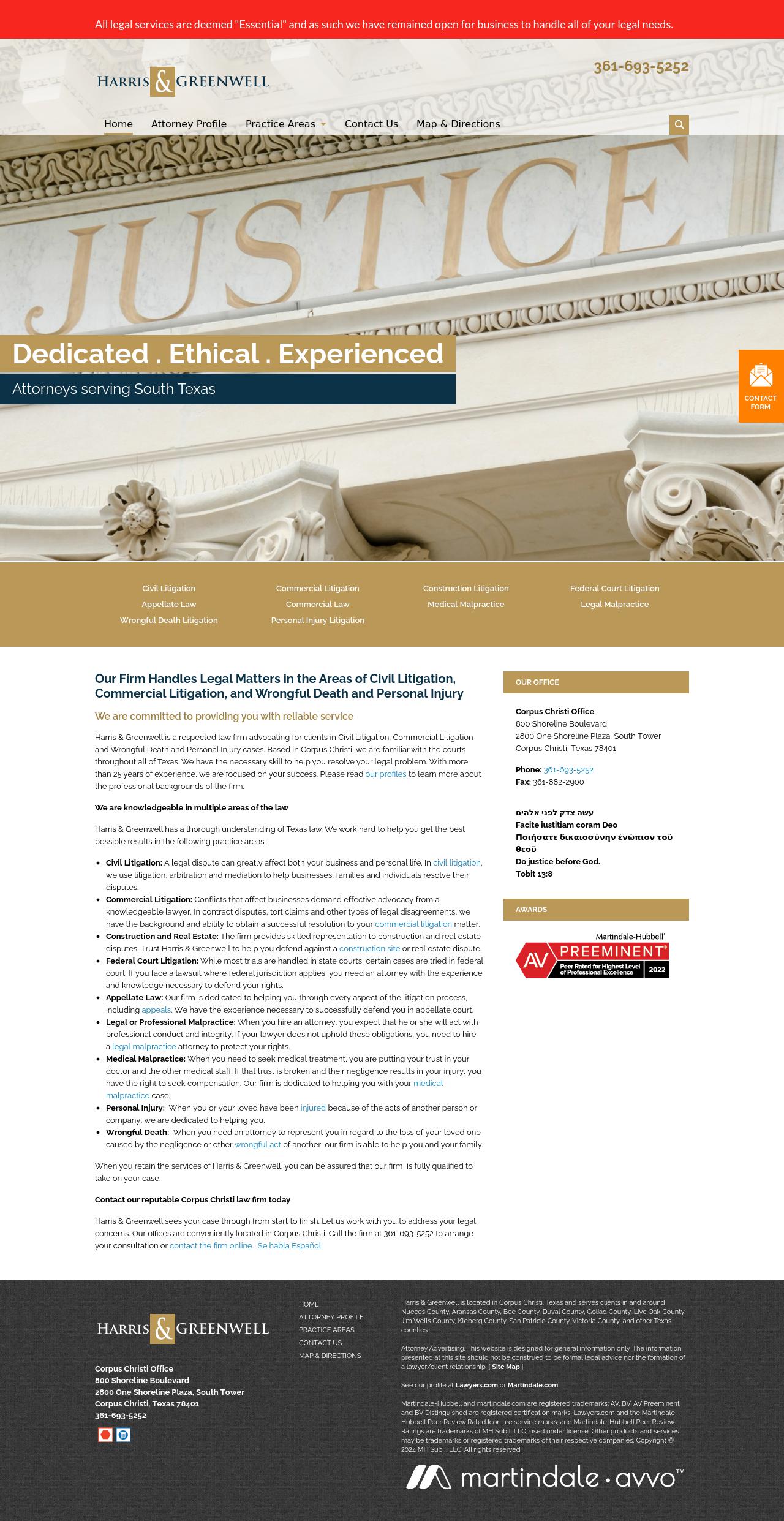This detailed caption describes the features and layout of the Harris and Greenwell attorney's office website. 

---

Screenshot of the Harris and Greenwell attorney's office website. In the top left corner of the webpage, the Harris and Greenwell logo is prominently displayed. The header spans the top of the page, featuring a bold red stripe with illegible white text due to the small font size. To the right of the logo is the firm’s contact number: 361-693-5252. Below the header, a navigation bar with several tabs shows the Home tab selected.

An image of a courthouse, with the word "Justice" inscribed above its entrance, adorns the webpage. Beneath this image, striking text reads, "Dedicated, Ethical, Experienced Attorneys Serving South Texas," clearly marking it as a professional legal services website.

Further down, the page offers a long promotional article detailing the firm's services. On the middle right side of the webpage, an emblematic red logo displays “AV” in white letters, with a red stripe at the top proclaiming “Preeminent,” signaling the firm’s high peer-reviewed rating.